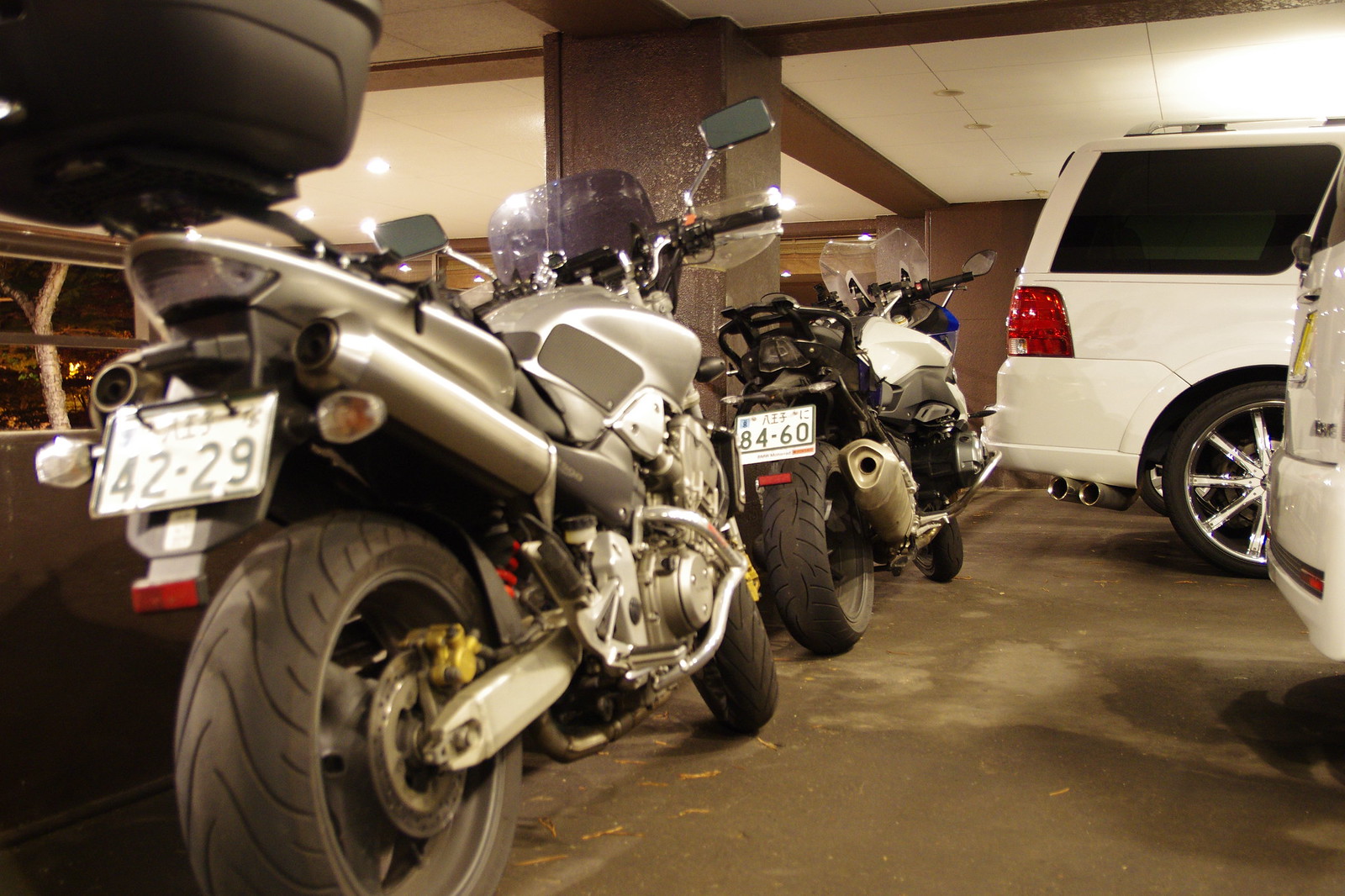The image captures the interior of a multi-storey parking garage scene dominated by two parked motorcycles which occupy most of the left side of the frame. The nearest motorcycle, positioned diagonally from the bottom left corner, is primarily metallic silver with dark gray wheels, two side mirrors, and a clear windshield. This bike has a license plate on its rear and resembles a street bike. Parked directly in front of it, the second motorcycle features a white and blue body with large, rounded black tires, a clear visor, and also has a license plate and two mirrors. To the right side of the image, partially visible, is the rear end of a large white SUV, presumed to be a Jeep due to its distinctive design, along with a slight glimpse of another white hatchback vehicle. The parking garage has a concrete floor with visible scratches near where the motorcycles are stationed, large structural supports, and a white and brown ceiling.